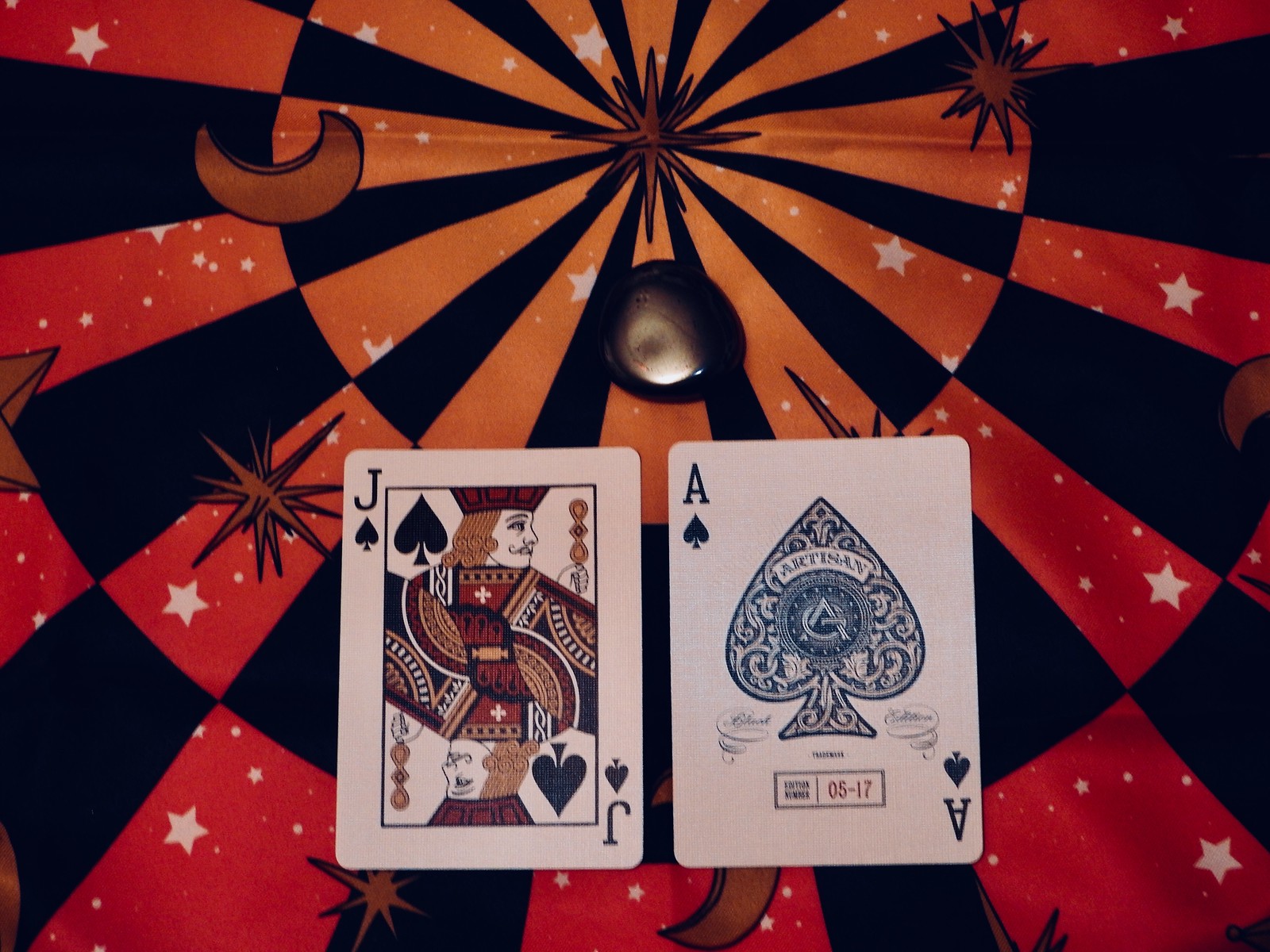The image features a richly detailed background comprised of concentric circular patterns in varying hues of blue, orange, and red. The innermost circle is formed by long, dark blue triangles interspersed with orange triangles, arranged around a central orange star. To the right of this star lies another orange star, while to the left is an orange moon. Surrounding this is another circular band of dark blue, highlighted with a slightly brighter shade of orange. Within this band, an orange star is located on the left side, and parts of another star and a moon are visible on the far left and right sides, respectively.

Encircling this, a third circle predominantly features deep blue and red triangles, adorned with small stars within the orange and red segments. In the foreground, two playing cards are displayed face-up: a jack of spades and an ace of spades. Beneath the jack of spades is a star, and beneath the ace of spades is a moon. Positioned above both cards is an object, possibly a stone, with a goldish hue and black edges. The intricate layering of colors and shapes creates a captivating visual composition.